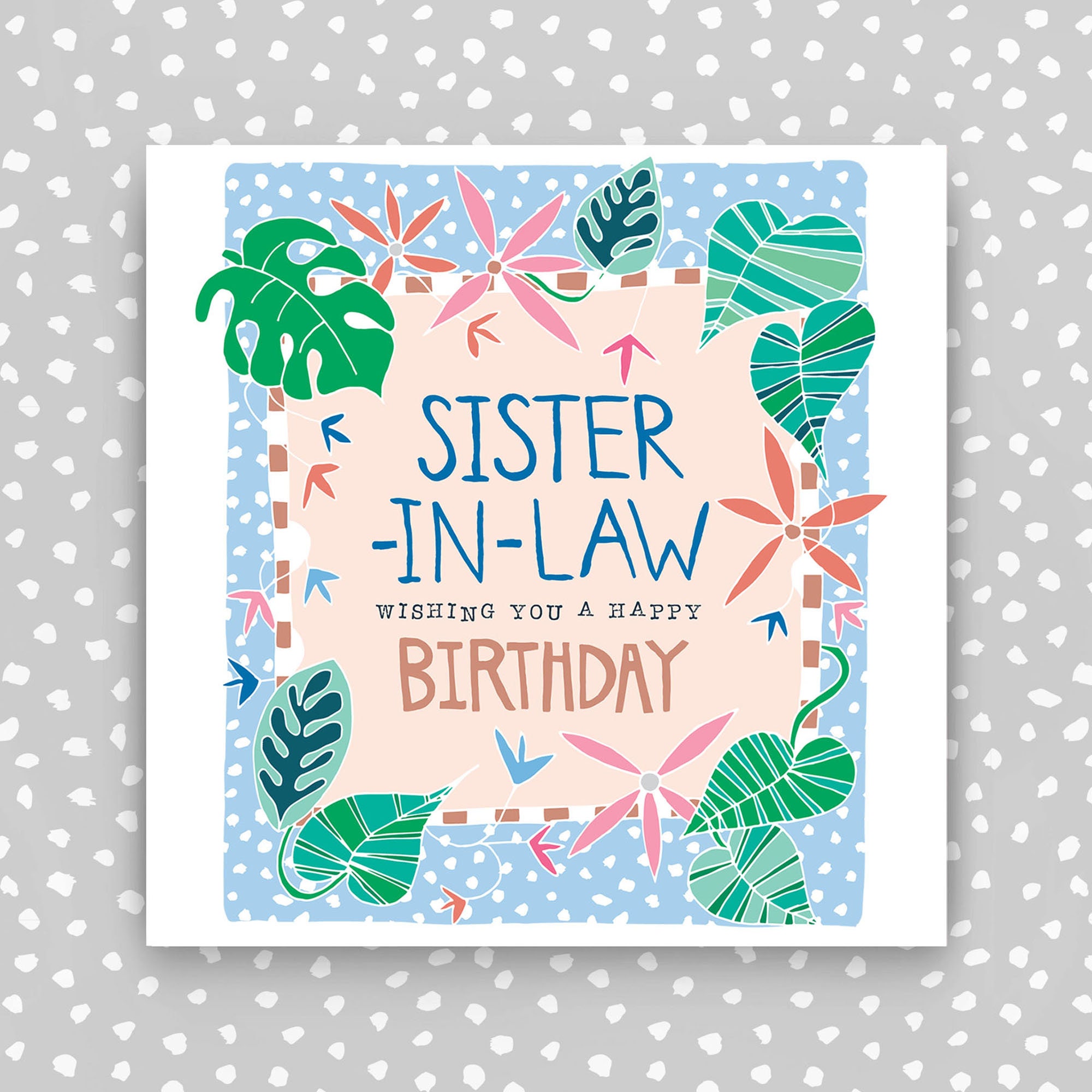This is an image of a birthday greeting card designed for a sister-in-law. The card is square and set against a textured backdrop of gray with white splotches. The card itself is white with an inner frame featuring an intricate design of green, blue, and pink leaves. There are also five-point flowers in shades of pink and orange, alongside multicolored arrows in blue, orange, and red. The text in the center reads "Sister-in-law" in large blue letters with "wishing you a happy" in smaller text and "birthday" in large text again, similar in size to "Sister-in-law." The text is set against a beige background, adding a subtle contrast and giving the card a beachy atmosphere. The white frame of the card also features a blue background dotted with white, adding to the layered, natural aesthetic.